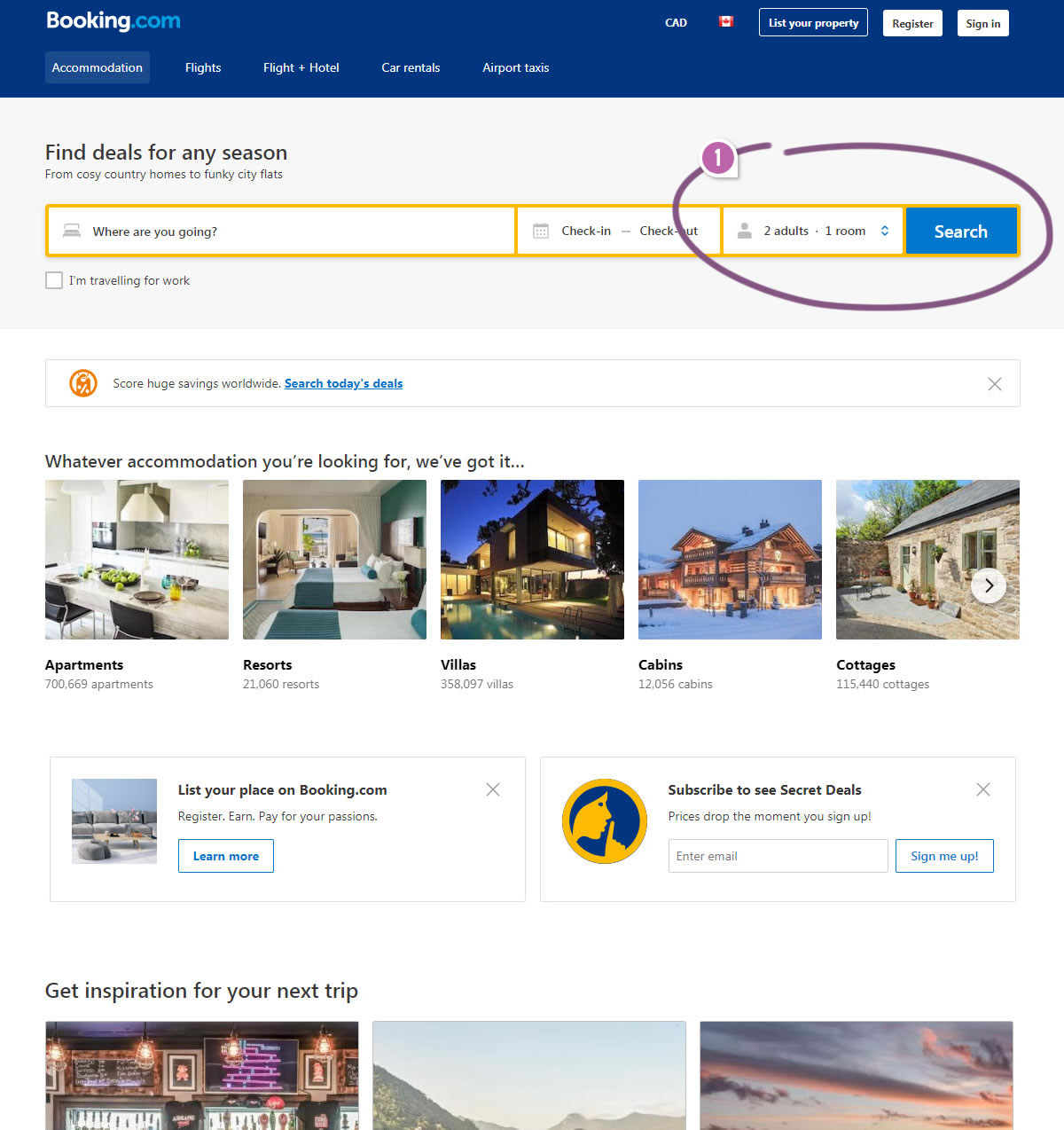This image is a screenshot from the website Booking.com. The top section features a prominent blue banner emblazoned with the Booking.com logo. Below this banner, there are several navigation tabs: "List your property," "Register," and "Sign In." Further down, there's an additional set of tabs for various services including "Accommodations," "Flights," "Flight + Hotel," "Car Rentals," and "Airport Taxis."

The main content area of the screenshot includes a white background header that reads "Find deals for any season," followed by a comprehensive search bar. The first field of the search bar prompts the user with "Where are you going?" where users can input their desired destination. Adjacent to this is the "Check-in" and "Check-out" section, allowing users to select their dates of stay. Highlighted by a purple circle, there is an option to specify the number of adults and rooms needed, set in this instance to "2 adults, 1 room." The blue "Search" button is prominently placed for users to initiate their search.

Below this search functionality, there is an optional checkbox with the label "I'm traveling for work" which can be ticked by users if applicable. Scrolling down further, the image showcases a selection of visual icons and thumbnails under the heading "Whatever accommodation you're looking for, we've got it," displaying various types of lodgings such as apartments, resorts, villas, cabins, and cottages.